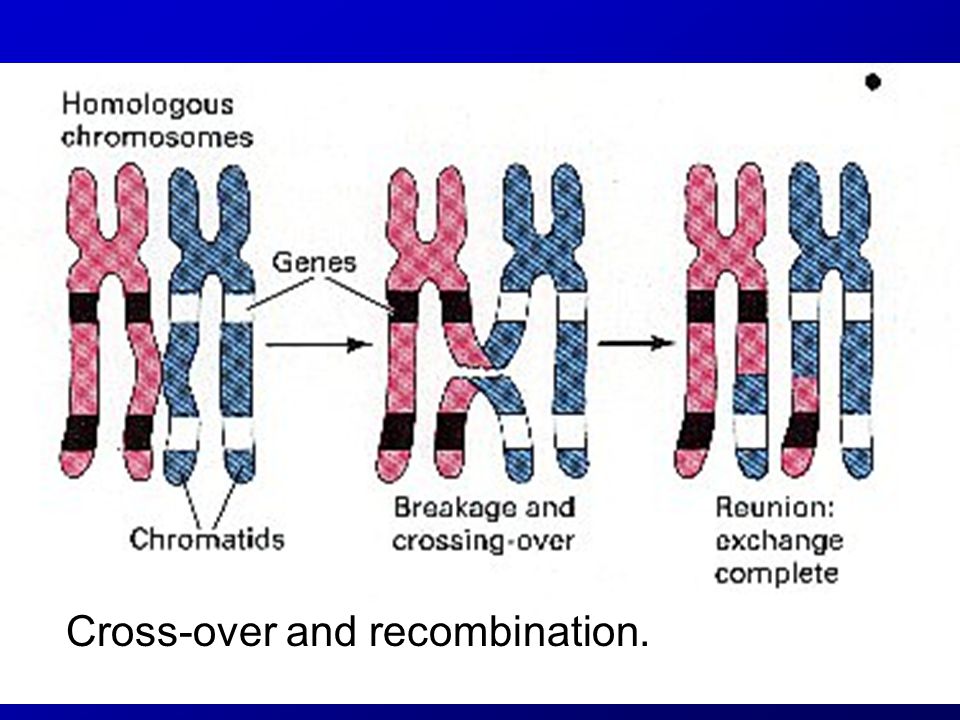This detailed infographic illustrates the process of crossover and recombination in chromosomes. Centered against a backdrop that could be reminiscent of an educational PowerPoint slide, the design features three sequential pairs of chromosomes, each represented with distinct color schemes: the left chromosomes are pink and the right chromosomes are blue. At the top, the title "Homologous Chromosomes" is prominently displayed to indicate the type of chromosomes shown.

The first pair, labeled simply as chromatids, introduces the homologous pairs. The second pair, labeled "Breakage and Crossing Over," visually demonstrates the exchange of segments between the chromatids, achieved through digital rendering. Finally, the third pair, labeled "Reunion Exchange Complete," shows the completion of the crossover process where the exchanged segments are integrated, color-coded in hues of red and blue interspersed with black or white cross sections, delineating the swapped genetic material.

The bottom of the infographic features large, bold, black text reading "Crossover and Recombination," summarizing the entire depicted process. Arrows guide the viewer's eye from the initial to the final stages, emphasizing the progression of genetic exchange. The infographic effectively communicates the key stages of genetic recombination in an educational setting.